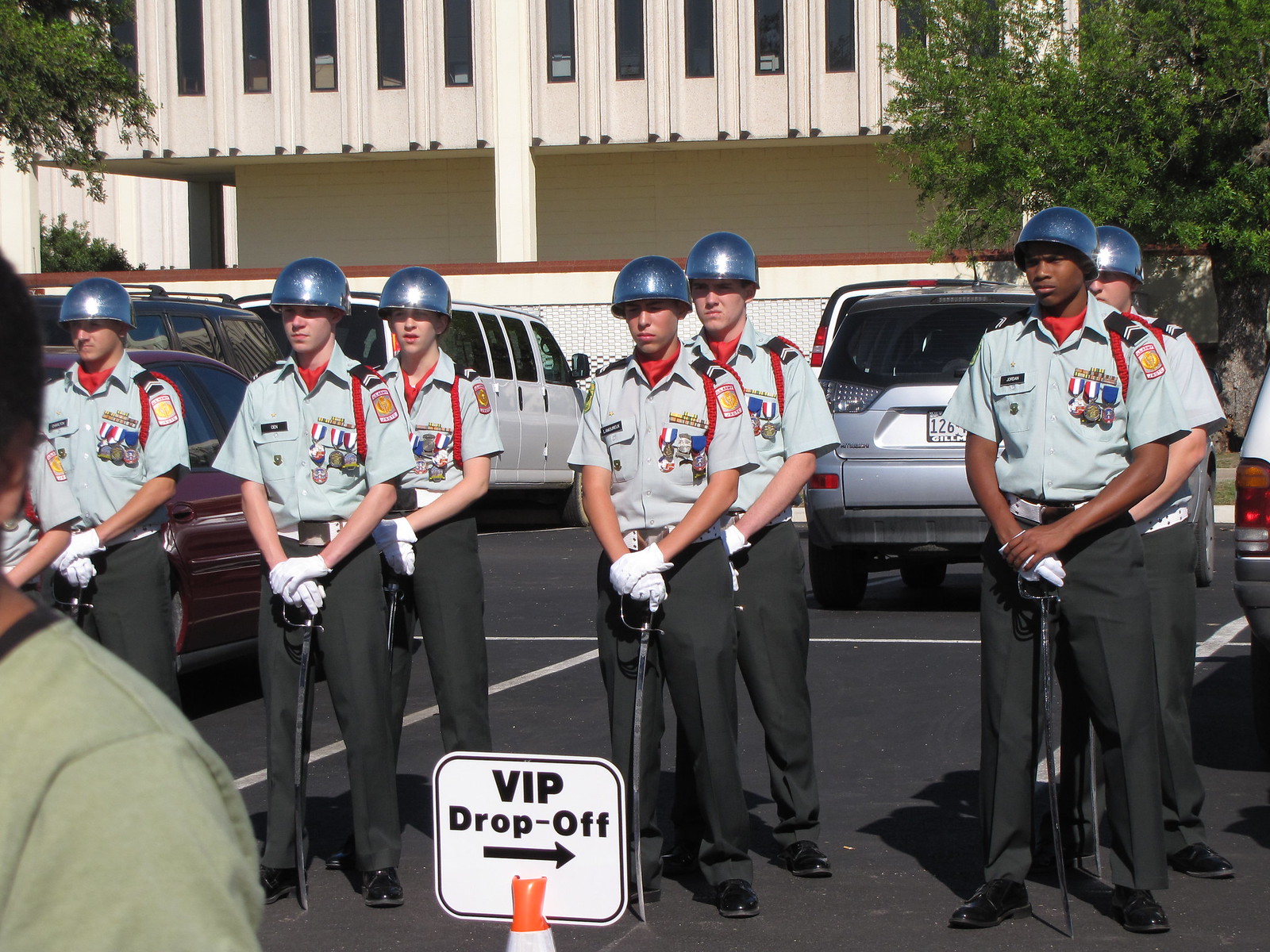The image depicts a disciplined formation of seven young security personnel or guards, captured in a color photograph with landscape orientation. They are standing outdoors in a parking lot in front of a large commercial building characterized by white stucco, long vertical glass windows, and flanked by trees on both sides. The men are arranged in neat rows, although the front left individual is partially cut off. Each guard is smartly dressed in a light blue short-sleeved shirt adorned with name tags, medals, and badges, coordinated with black or dark gray trousers and white gloves. They wear matching blue helmets and sport red scarves around their necks. They hold ceremonial swords, the blades pointed down to the ground, as part of their regimented posture. A white sign with black lettering reading "VIP drop-off" with an arrow pointing to the right is prominently positioned in the lower center of the image. In the background, several parked vehicles, including a limousine, are visible. A green-shirted individual is partially seen on the bottom left corner, adding a touch of activity to the otherwise orderly scene.